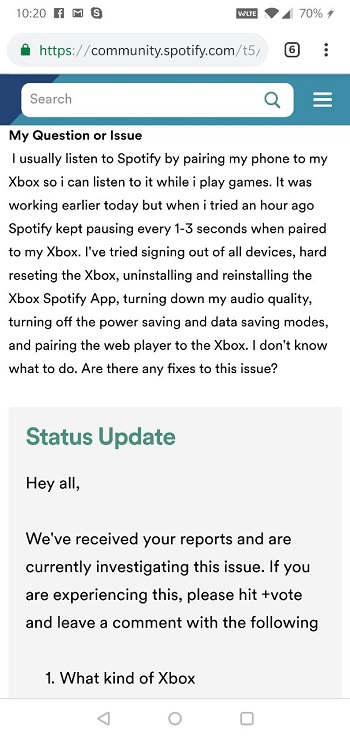This image depicts a screenshot set against a white background. In the upper left corner, the time is displayed in light gray, reading 10:20. To the right of the time are two icons: one for Facebook and the other for Gmail. The upper right corner shows a battery icon with a 70% charge.

Below these elements is the address bar. It displays "HTTPS" in green text followed by "community.spotify.com" in dark gray text, indicating a secure connection to the Spotify Community website. Below the address bar, there is a blue banner containing a white search bar.

Further down, bold black text reads "My question or issue." Under this heading, there is a detailed description of a problem: "I usually listen to Spotify by pairing my phone to my Xbox so I can listen to it while I play games. It was working earlier today, but when I tried an hour ago, Spotify kept pausing every 1-3 seconds when paired to my Xbox."

Below this issue description, there is a gray box with dark green bold text that reads "Status Update."